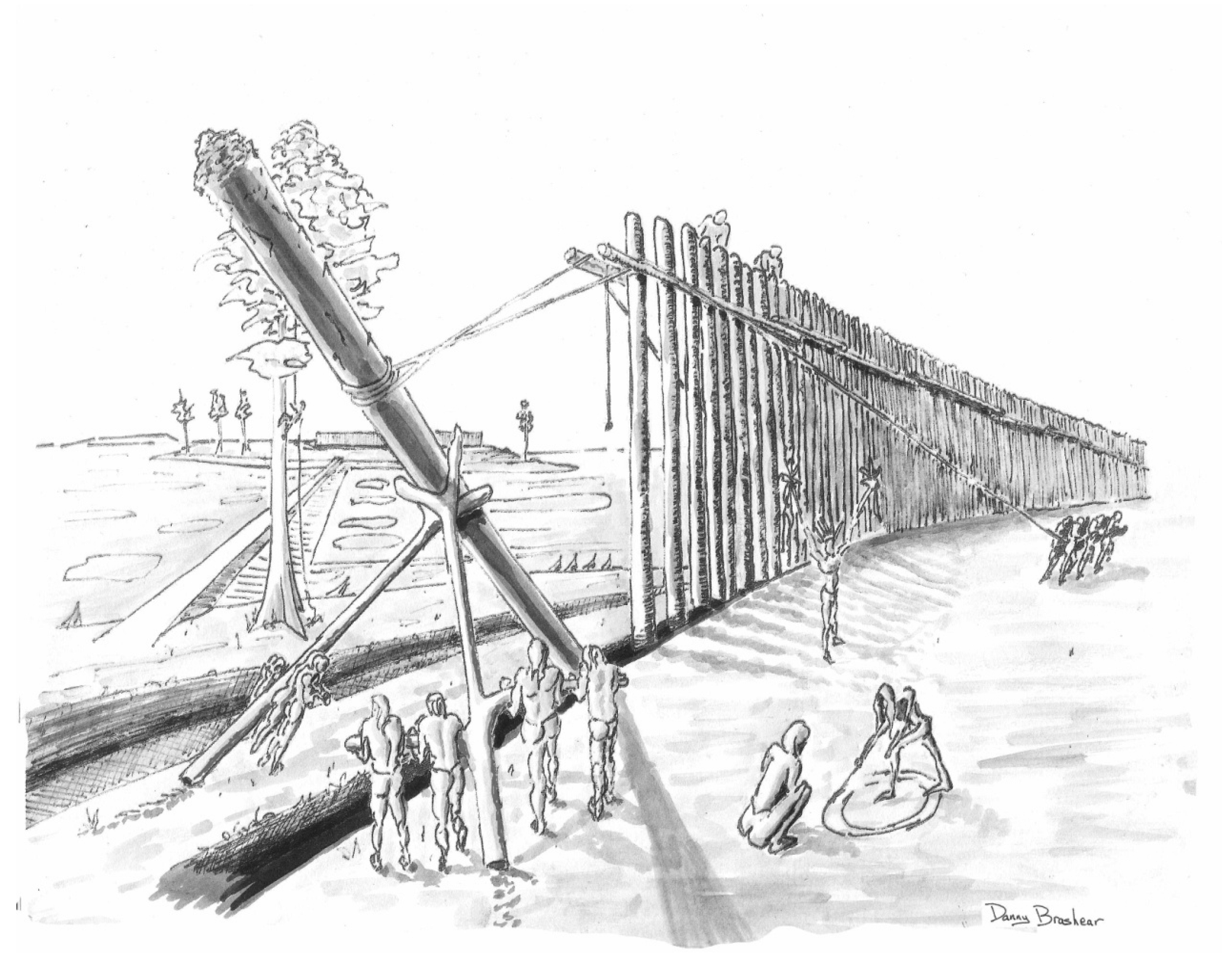This is a highly detailed, black and white pencil drawing by Danny Broder, as indicated by the signature in cursive at the bottom right corner. The artwork vividly depicts an ancient scene where numerous individuals are working together to erect an enormous wooden fence. Central to the image are several groups of men, all wearing loincloths, skillfully hoisting giant logs and using lever systems to position each post into place. They appear to be utilizing pieces of wood with V-shaped tops to push the heavy logs upright. 

In the background, behind the nearly completed section of the fence, there are trees and an open field, possibly indicating the expanse of land they intend to encircle. Additionally, towards the left side of the image, there is what seems to be a statue adjacent to a walkway leading down to the construction area. Among the workers, a person is seen orchestrating the efforts, directing the groups efficiently. Off to the side, two other individuals are intently focused on plans, likely determining the layout of this massive circular fence intended to surround their land.